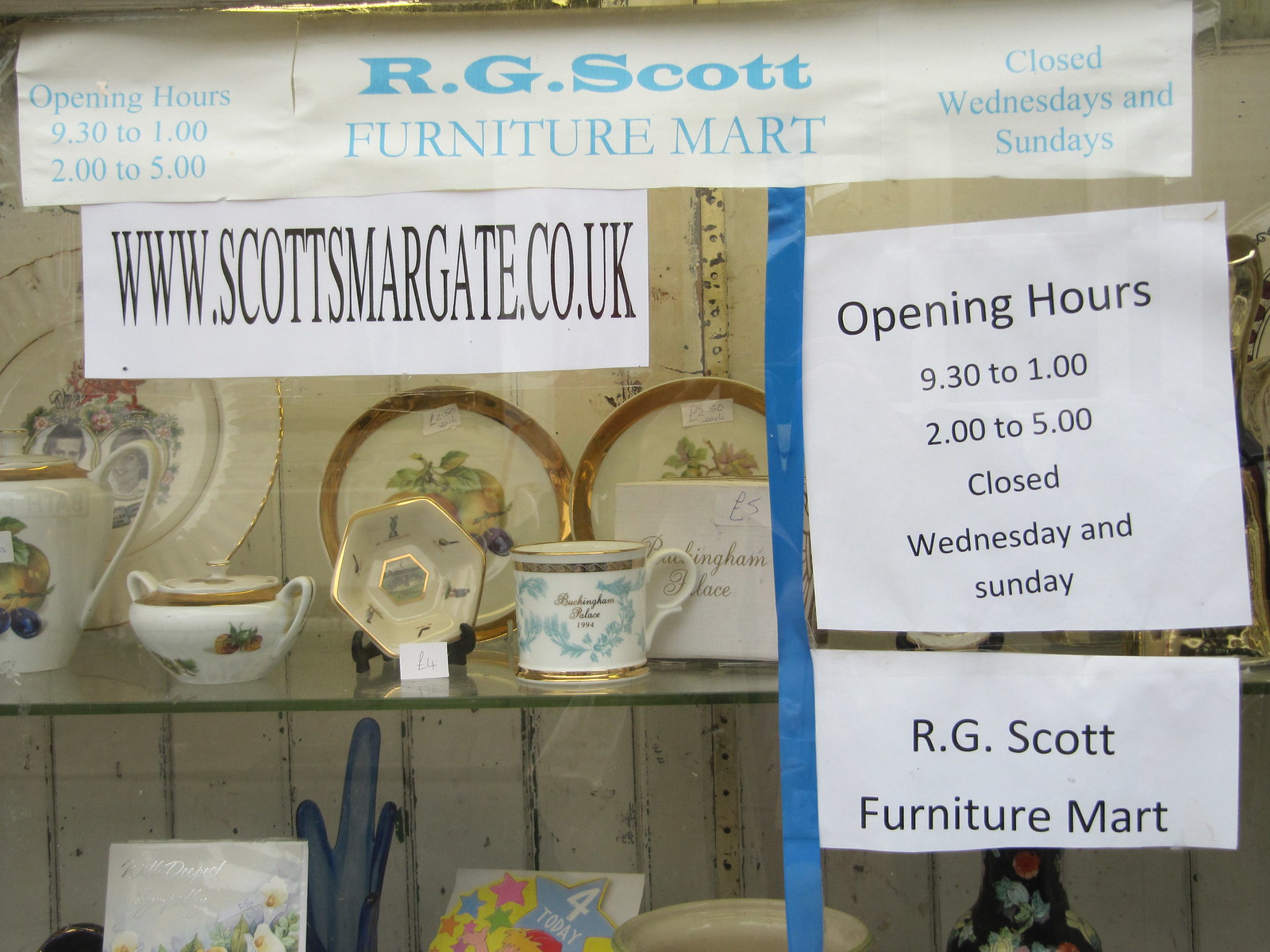The image depicts a storefront display showcasing a glass shelving unit filled with an assortment of decorative dishes, cups, and containers. The shelves are enclosed with glass windows, and prominently displayed at the top are multiple signs for "R.G. Scott Furniture Mart," listing the opening hours (9:30 AM to 1:00 PM and 2:00 PM to 5:00 PM, closed Wednesdays and Sundays), and the website www.scottsmargate.co.uk. The displayed items are predominantly white with elegant gold rims and feature various patterns, including flowers and fruits. A large plate with a central design and gold trim is positioned on the left side, alongside smaller similarly adorned plates. Notable objects include a gravy boat, an ashtray on a stand, and a cup adorned with blue flowers and gold trim. Below the shelf, there is art, possibly blown glass, and a couple of cards, one resembling a birthday card. The setting appears to be indoors, likely a used furniture store, captured during closed hours. The colors throughout the display include white, gold, blue, green, black, yellow, and light blue.